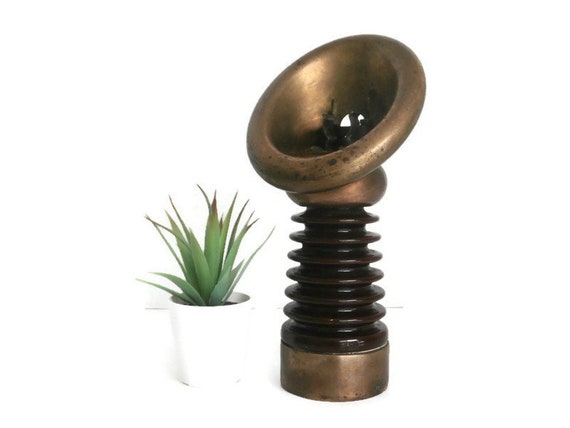The image features a unique corkscrew-like object with a distinctly crafted design. The top of the item is round, resembling a small bowl with an inner cavity and a central hole. This part, as well as the bottom, appears to be made of metal, giving off a bronze-like sheen. The bottom section extends into a corkscrew shape, primarily brown in color, and is anchored by a round base.

In the background to the left, there is a cup filled with soil and hosting a slender, green, pointed plant. The juxtaposition of the metal corkscrew object and the organic plant creates an interesting contrast within the scene.